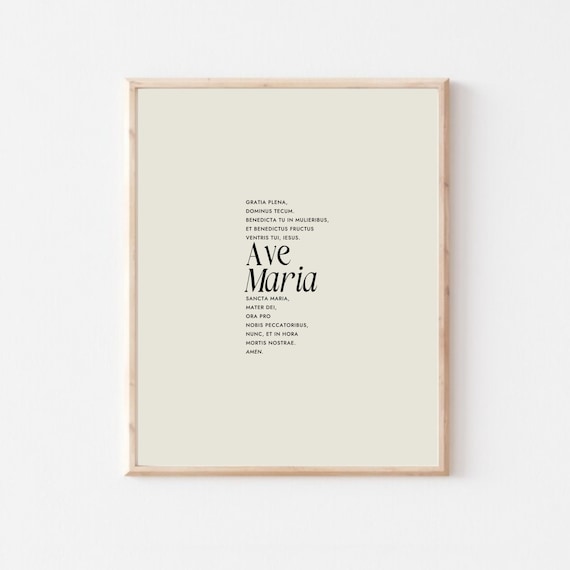This image depicts a framed wall canvas on a white wall. The frame is made of light-colored wood and encloses a cream-colored canvas. In the center of the canvas, the title "Ave Maria" is prominently displayed in large, bold black letters. Surrounding the title are the lyrics to "Ave Maria," which are printed in smaller, yet equally bold, black letters. The text consists of varying line lengths, with five lines above and about seven lines below "Ave Maria." The words appear to be in Latin, including phrases like "Santa Maria, Mater Dei, Ora Pro Nobis Peccatoribis, Nunc et in Hora Mortis Nostrae. Amen." Overall, it's a simple yet elegant presentation of this classic prayer, meticulously arranged on the canvas.